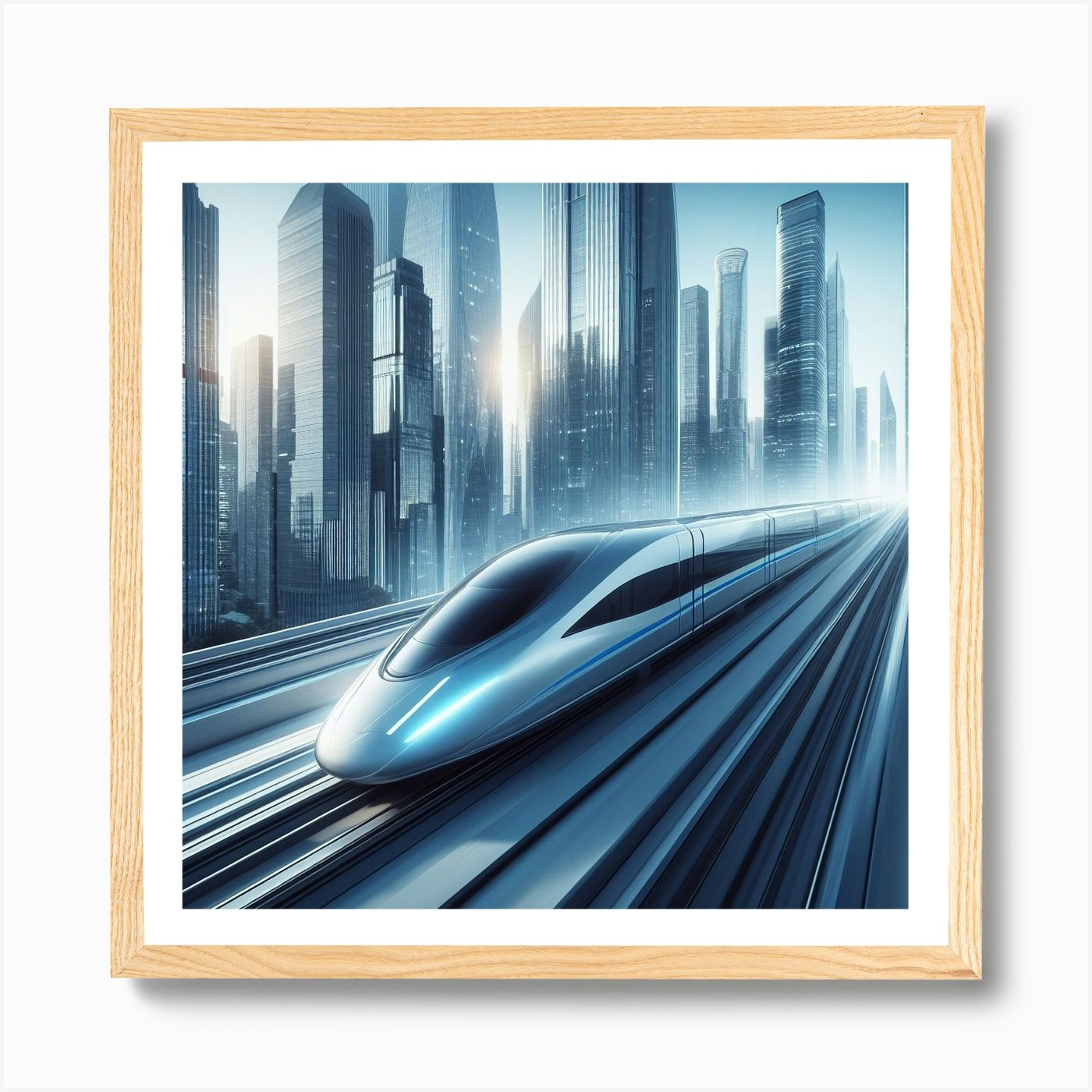The image is a captivating sci-fi digital artwork set within a light wood grain square frame with a white matte border. The art features a sleek, futuristic high-speed train, likely a bullet train, with a narrow, aerodynamic, triangular-shaped nose. The train's silver body is accentuated by a blue line running along its side, and its dark-tinted, oval window at the front adds to its modern appeal. The painting uses a monochromatic color palette dominated by blues and whites, enhancing the sense of speed and futurism. In the background, there's a city skyline with numerous bluish, glass-like skyscrapers, which further emphasizes the overall blue theme. The buildings reach upwards, with the sun's rays piercing through the gaps between them, creating a dynamic interplay of light and shadows. There's a subtle blur effect beneath the train, suggesting its high velocity. The entire piece is illuminated from the upper left, casting a drop shadow to the right of the frame, adding depth and dimension to the artwork.